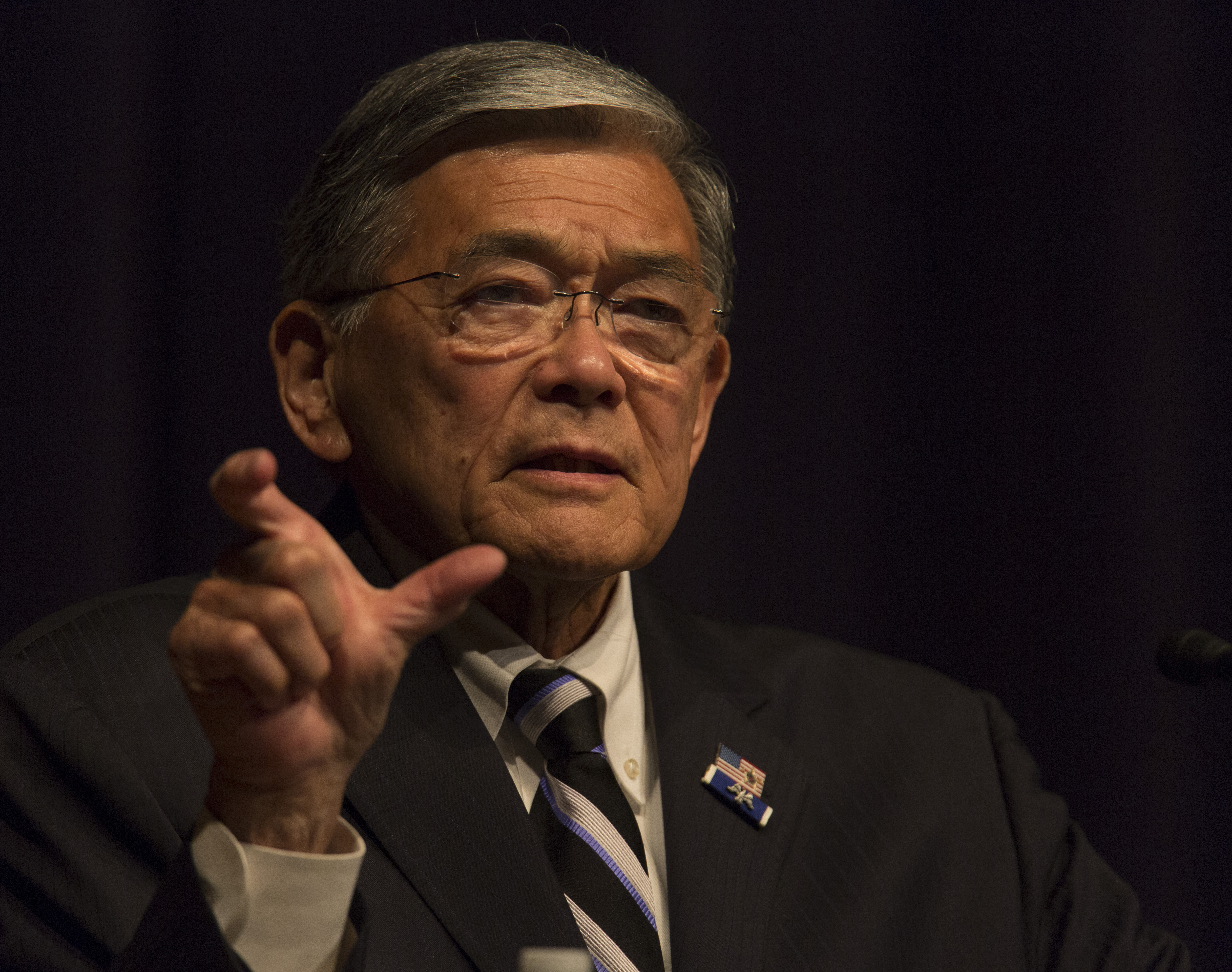The image depicts an elderly white male with grey-white hair styled in a side parting. He is wearing frameless glasses with a soft square shape and has a serious expression on his face. Dressed in a dark-colored suit jacket, he also sports a white dress shirt with the collar buttoned down and a dark tie decorated with white and light blue diagonal stripes. On the left lapel of his jacket, there is an American flag pin featuring red and white stripes with a blue rectangle and a gold insignia. Below that, another pin displays a blue band featuring a metallic bird. The man is posed with his right hand raised, his thumb and index finger forming a claw-like shape, as if measuring something. The background is entirely black, emphasizing the subject's serious demeanor and attire.